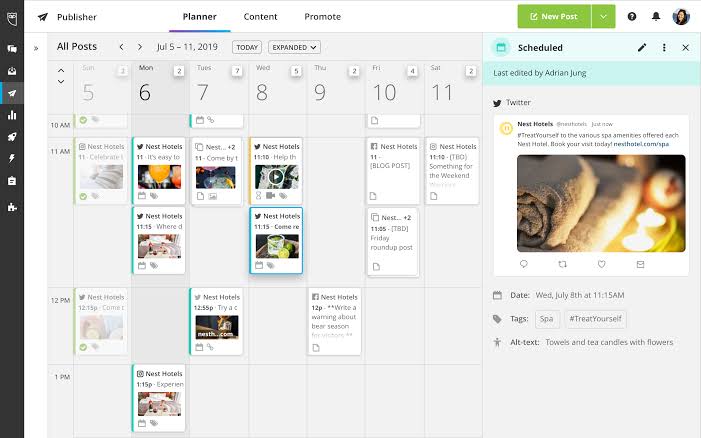The image showcases a planner page displayed on a laptop. The background is a light gray, while the interface includes a prominent white border along the top and the inner left side. The far left side features a vertical black border with icons aligned down its length.

At the top of the page, a horizontal banner presents several sections: "Publisher," "Planner," "Content," and "Promote." On the far right of this banner is a rectangular green drop-down menu labeled "New Post" in white text. Directly beneath this banner is a navigation bar where "All Posts" is displayed on the left, followed by directional arrows pointing left and right, and a date range from "June 5th through 11th, 2019."

Within a section marked by an outlined rectangle, there is black text reading "Today." Next to it, another outlined rectangle contains the word "Expanded" alongside a drop-down menu. Towards the far-right, the word "Scheduled" is visible.

Beneath this section, it indicates that the last edit was made by "Adrienne Yong." Further down, the words "Twitter" are shown, followed by a tweet regarding "Next Hotels."

At the bottom of the planner page, there's a horizontal calendar extending from Sunday to Saturday, displaying scheduled posts for "Nest Hotels" on each day. Each day within the calendar contains its own individual picture to represent the respective post.